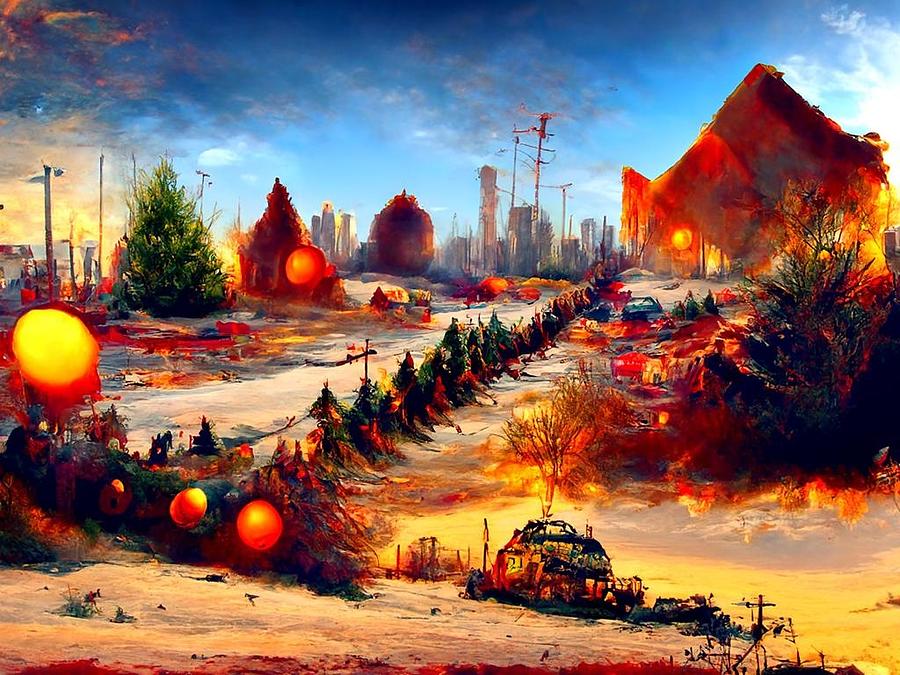This vivid, abstract painting presents a surreal, post-apocalyptic landscape. The scene is marked by a desolate yet colorful atmosphere, dominated by a vibrant blue sky with scattered clouds. Cutting across the image diagonally is a line of what appear to be evergreen trees, leading the eye from the lower left to the upper right, giving an illusion of depth and direction. These trees, reminiscent of Christmas trees, juxtapose the chaotic background.

The background features a cityscape silhouetted against the sky, with tall, spindly structures that could be buildings and utility poles. Particularly striking are several large, fiery orange globes scattered throughout the scene, with some resembling triangles or diamonds, enhancing the fantastical nature of the image.

Towards the front, the ground morphs into a barren, almost desert-like expanse, littered with what looks like a burnt-out car and a flaming tree nearby. The remnants of buildings reduced to ashes contribute to the overall sense of abandonment and destruction.

On the right side of the painting, intermixed with the trees, are curious elements like a large evergreen and another tree seemingly bearing an oversized orange. Adding to the surrealism are large, lemon-like shapes protruding from the left. These bizarre, almost fruit-like objects appear to be aflame, reflecting the painting's unsettling and chaotic vibe.

The painting masterfully combines a bright palette with ominous, fiery elements, creating an eerie yet captivating vision of a devastated world, each detail adding to its rich tapestry.